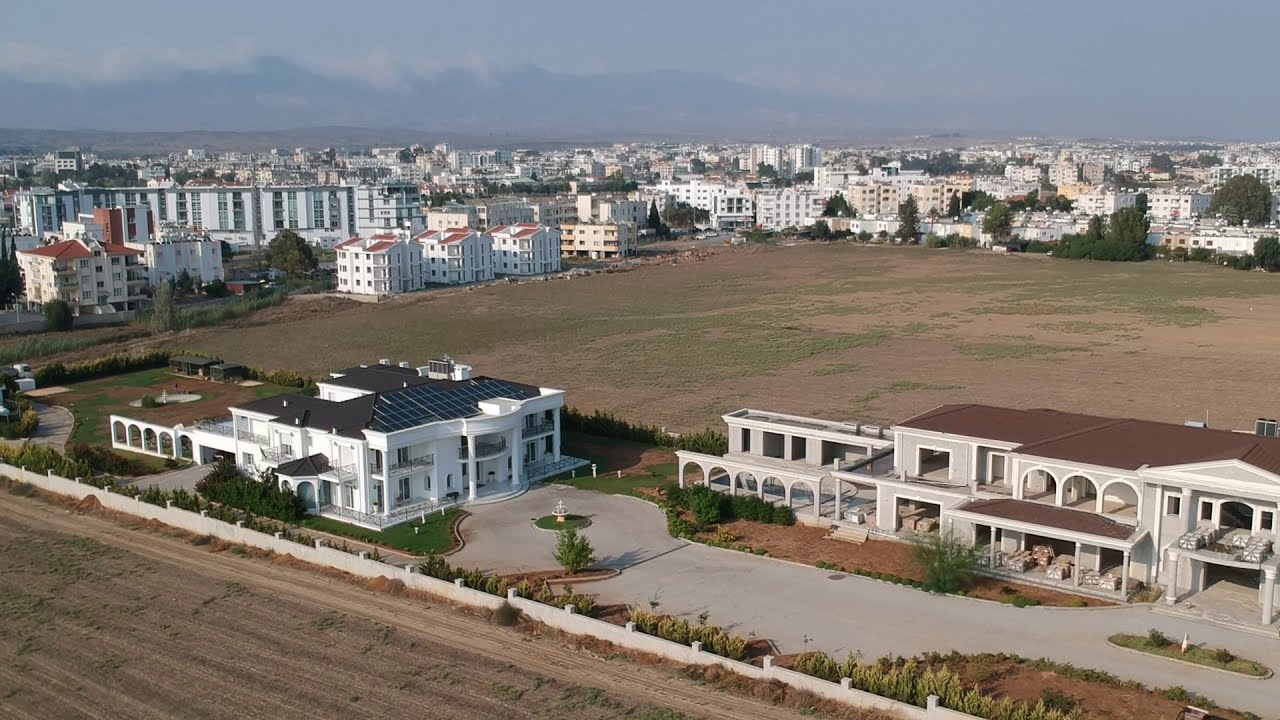In the foreground of the image, there are two luxurious buildings separated by a circular driveway with a fountain at its center. To the left, a large white two-story building with solar panels on the roof, enclosed by a stone wall, exudes an air of exclusivity. Ahead of these is a large gray building with a brown rooftop and intricate arched windows, possibly a hotel, with a sprawling sidewalk in front. These buildings stand out, isolated within a vast expanse of dirt and sparse grass that forms a square in the middle of the scene.

Surrounding this open area and filling the background is an extensive array of densely packed residential structures. The majority of these buildings are white, sporting red rooftops, and consist of apartment complexes and condominium units, creating a striking contrast with the openness of the foreground. Further into the distance, low-lying mountains softly rise against a sky that is a blend of light blue and gray, studded with clouds. The entire scene reveals a juxtaposition of opulence against a backdrop of crowded urban living, hinting at a bustling city landscape possibly in a foreign country. There is no text in the image, allowing the intricate details of the buildings and landscape to speak for themselves.